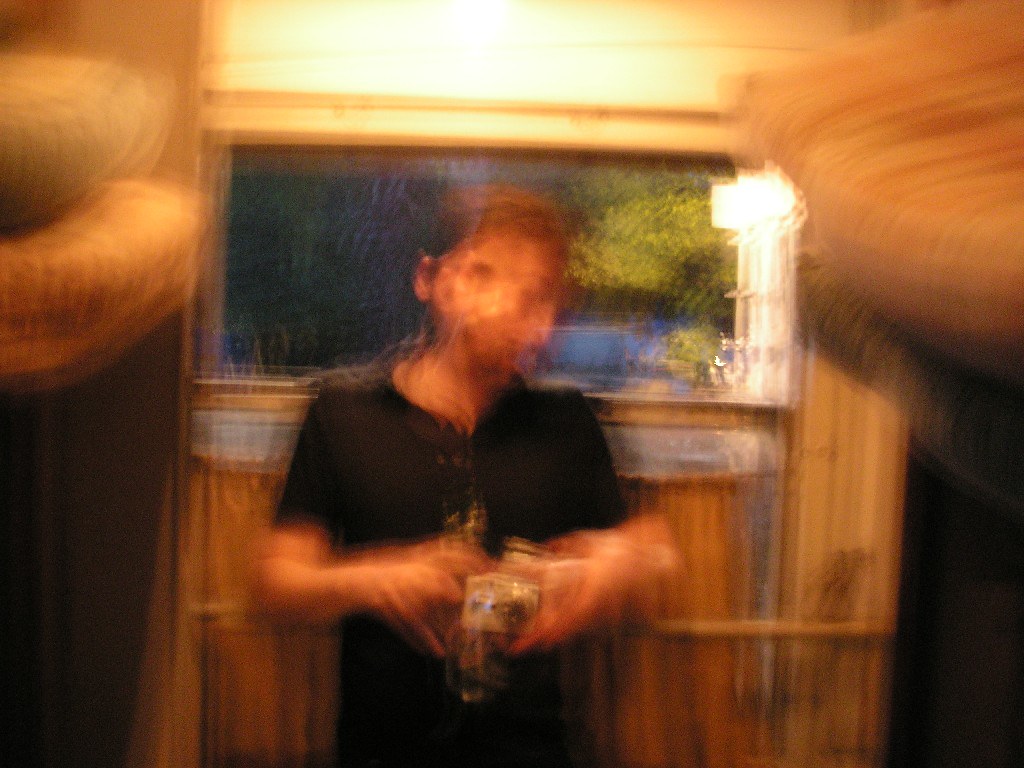The image is an extremely blurry photograph of a man with short brown hair and a pale to medium skin tone, who is standing with his head slightly tilted to the left, facing the camera. He is wearing a short-sleeved black shirt and holding an indistinct object in both of his hands near his chest. In the background, there appears to be a window or a painting depicting a blue sky and green foliage, possibly a shrub or tree, against a brown wall. The upper part of the photo is notably brighter, indicating that a flash may have been used or there is strong lighting in the room. Additionally, on either side of the frame, there are vaguely discernible rounded objects attached to the wall, with the object on the right protruding slightly more. A pipe or tube can also be seen running along the wall behind the man's back. The overall lack of focus and detail makes the exact elements and context of the image difficult to determine.